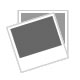This image showcases a plain sage green t-shirt, most likely designed for a product page, given the clean and empty white background akin to a PNG image. The medium to large-sized shirt is highlighted by its short sleeves and traditional neckline, suggesting it could be a man's t-shirt. The fabric exhibits some natural creases and folds, enhancing the realistic depiction. Dominating the chest area is a vintage police car graphic, stylized as an outline drawing in white, allowing the green hue of the shirt to peek through. The classic car, reminiscent of early 1900s police vehicles, features a small, old-fashioned single siren on the roof, as well as discernible details like tires and other car markings. Additionally, there's a tiny, somewhat indistinct white logo resembling a fish located on the left sleeve, presumably representing the brand.